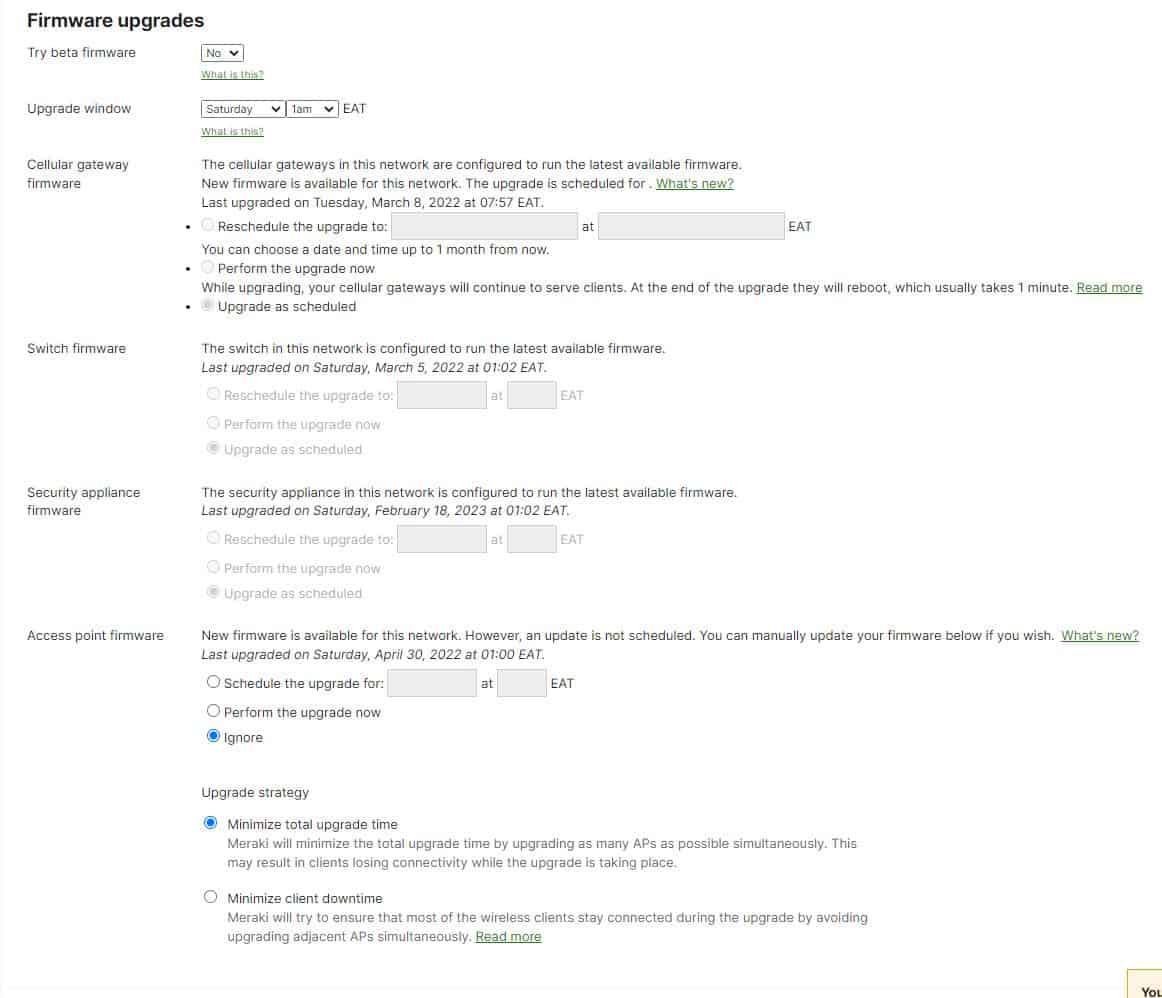**Image Description: Detailed Firmware Upgrade Settings Page**

The image showcases a comprehensive firmware management interface, composed of black text on a white background. In bold black letters at the upper left corner, the heading "Firmware Upgrades" is prominently displayed.

On the left side of the page, various section headings are listed, corresponding to detailed settings on the right. The first section is titled "Try Beta Firmware" and features a toggle switch with options to select 'Yes' or 'No'. Beneath it, a hyperlinked line labeled "What is this?" provides additional information.

The following section is "Upgrade Window," with a drop-down menu allowing the selection of specific days and times for firmware updates. Another green hyperlink, also labeled "What is this?" offers more details on this setting.

Next, under "Cellular Gateway Firmware," the status on the right informs that the cellular gateways in this network are set to operate on the latest available firmware. This is supplemented with further technical details.

For the "Switch Firmware" section, it states that the switches are configured to run the latest firmware, noting their last upgrade occurred on Saturday, March 5th, 2022, at 1:02 EAT.

Similarly, the "Security Appliance Firmware" section confirms that the security appliances are also configured with the latest firmware, reflecting the same upgrade date.

The "Access Point Firmware" section advises that new firmware is available yet unscheduled for update. A blue radio button marked 'Ignore' is selected. Below this, "Upgrade Strategy" presents two options: 'Minimize Total Upgrade Time,' which is turned on (indicated by a blue radio button), and 'Minimize Client Downtime,' which is not selected.

This detailed interface demonstrates the extensive configurations available for managing firmware across various network devices.